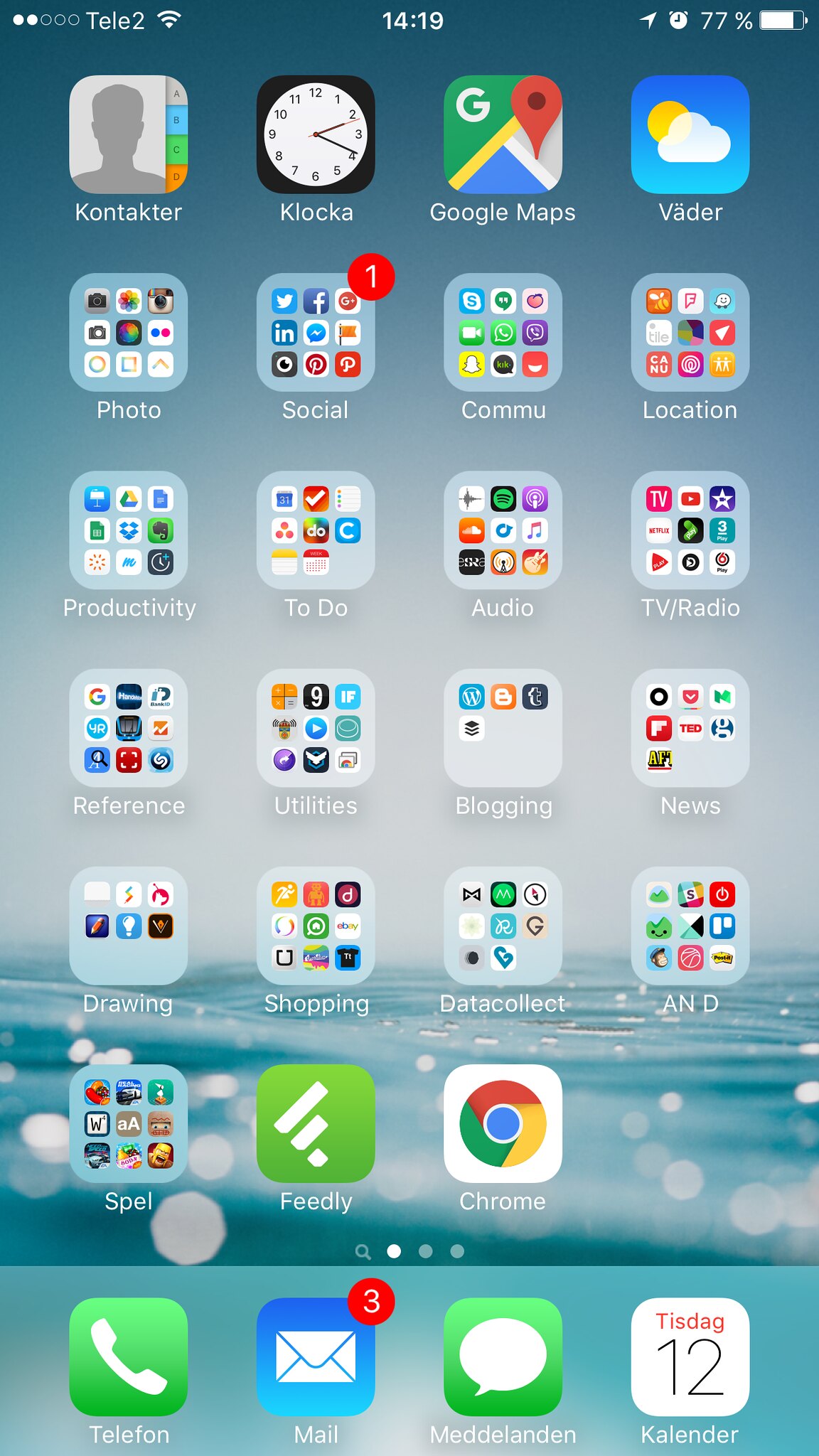This image is a detailed screenshot of an iPhone home screen.

At the top portion of the screen, several status icons are visible:
- The cellular signal shows two out of three bars.
- The carrier name displayed is "TELA 2."
- The Wi-Fi signal is at full strength.
- The time is 14:19.
- The location services icon is active.
- An alarm clock icon indicates that an alarm has been set.
- The battery percentage is at 77%.

The wallpaper features a serene scene with a grayish-blue sky and a greenish-blue body of water.

The home screen is organized with numerous app folders, some labeled in another language:
1. "Kontakter" (Contacts)
2. "CLOCKA" (Clock)
3. "Google Maps"
4. "Väder" (Weather)
5. "Foto" (Photos)
6. "Social" (Social media apps)
7. "Kommunikation" (Communications)
8. "Plats" (Location-based apps)
9. "Produktivitet" (Productivity)
10. "Ljud" (Audio)
11. "TV"
12. "Radio"
13. "Referens" (Reference)
14. "Verktyg" (Utilities)
15. "Bloggning" (Blogging)
16. "Nyheter" (News)
17. "Ritning" (Drawing)
18. "Shopping" (Shopping)
19. "Datainsamling" (Data Collection)
20. "E&D"
21. "Stavning" (Spelling)

In addition to these folders, there are individual app icons:
- "Feely"
- "Chrome"

The dock at the bottom of the screen contains four essential apps:
- "Telefon" (Telephone)
- "Mail"
- "Meddelanden" (Messaging)
- "Kalender" (Calendar)

This home screen is meticulously organized, with folders grouping related apps together, providing a streamlined user experience.